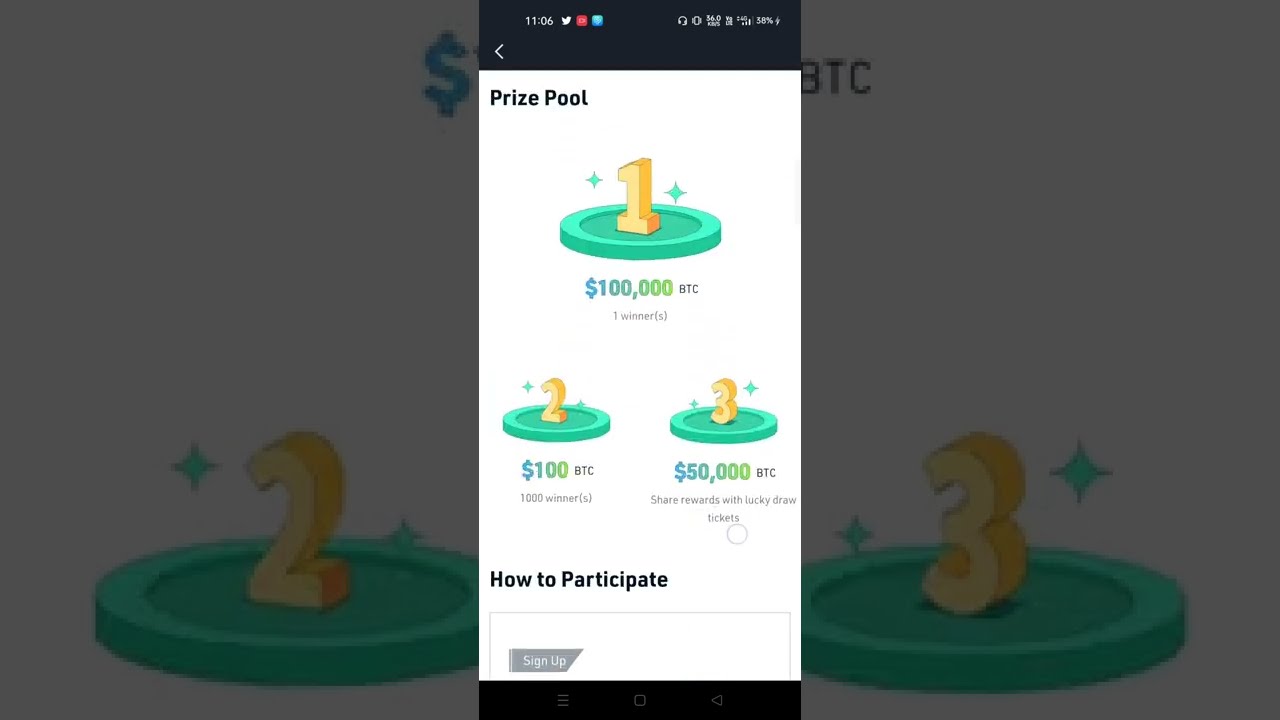This image, a horizontal rectangular screenshot from a cell phone, displays a promotional page for a game. At the top, the status bar shows the time "11:06" along with some icons indicating battery level and other notifications, though they are blurred and hard to read. The main content of the page has a white background and is centered, with "Prize Pool" written at the top in bold black letters.

Below the heading, three green circular bases are prominently displayed, each crowned with a gold 3D numeral indicating the ranking of the prizes. The first place prize, shown on the left, features a golden "1" above the amount "100,000 BTC," indicating one winner. The second prize, in the middle with a gold "2," offers "100 BTC" to one thousand winners. The third prize, on the right with a gold "3," promises "50,000 BTC" as shared rewards with lucky draw tickets.

At the bottom of the image, the text "How to Participate" appears in black, followed by a sign-up button. To the left and right of the central content are close-up views of the gold "2" and "3" numerals on their green bases. The overall design has a darker border that transitions into the lighter center, emphasizing the central information.